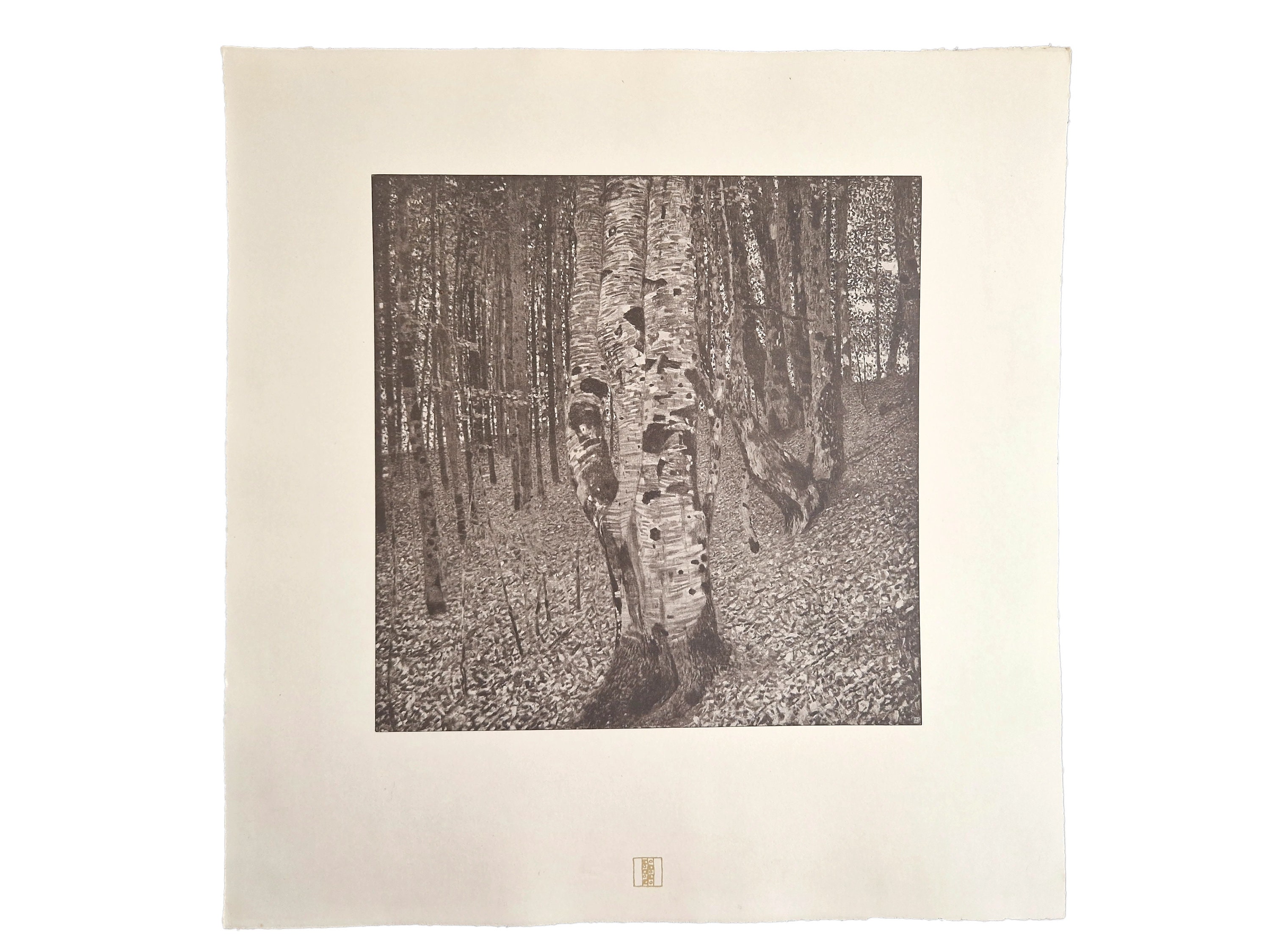The black and white photograph captures a dense forest scene, characterized by its numerous thin tree trunks stretching upwards on a gentle hillside. The stark monochrome palette enhances the textured details of the forest floor, which is strewn with fallen leaves from the hardwood trees. Dominating the foreground is a peculiar, thick-trunked tree, distinguished by multiple large branches that sprout vertically from its base and a series of organic black and white stripes, reminiscent of zebra patterns. This primary tree is further marked by numerous holes, likely created by animals inhabiting the decayed wood. The overall image, set within a beige matting, presents a clear and brightly lit vista, with the bright sky visible through the upper portions of the densely packed trees.